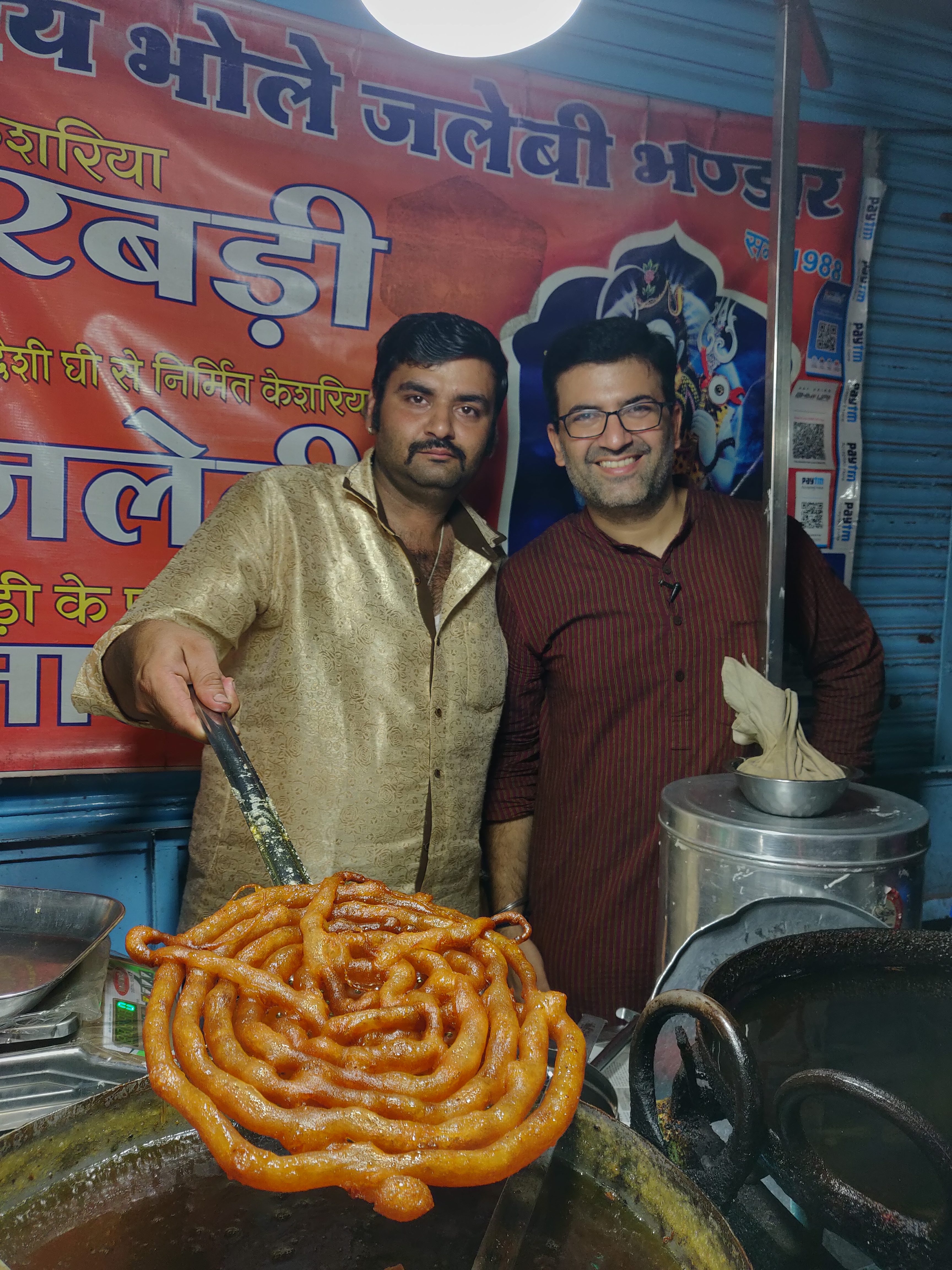In this detailed photographic image, two Middle Eastern men are standing close to each other, seemingly indoors near a cooking stand. The man on the right, who is smiling, has a darker complexion with black hair, glasses, and a subtle mustache and beard shadow. He is dressed in a long-sleeve maroon button-up shirt with white stripes. To his left is a man with black hair and a prominent black mustache, clad in a shiny, golden long-sleeve collared shirt. He is holding a large spatula, presenting a beautifully fried, spiral-shaped dough item, likely a traditional Middle Eastern or Indian delicacy. 

In front of them is a large pot of oil where the food is presumably being fried. Also visible is another black pot and a silver container that likely holds more dough. The background features an orange sign with non-Roman characters, possibly Middle Eastern or Indian writing, further accentuating the cultural setting. A light illuminates the man in the foreground, highlighting their culinary activity and the intricate details of their attire and surroundings.